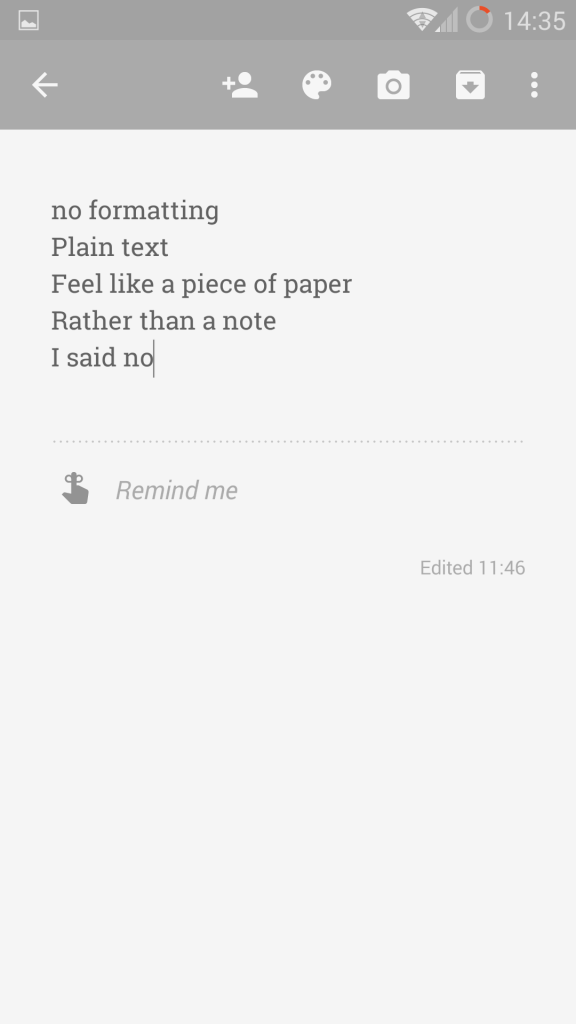This is a detailed screen capture of a smartphone interface, most likely showcasing a note-taking application characterized by its utilitarian design with a grayscale color scheme. At the top of the screen, there is a horizontally oriented, two-tone gray bar. Situated in the upper left corner of this bar, there is a white icon representing an image. On the upper right side, several white icons are visible: a triangular Wi-Fi signal symbol, which indicates the Wi-Fi strength as one bar out of four, a gray circle positioned at the one o'clock mark with a small red notification dot, and the time, 1435, displayed in white digits.

Beneath this bar, a row of white icons is laid out on a gray background, including a left-pointing arrow, an add contact icon, a paint palette icon, a camera icon, and a file download icon with three vertically aligned white dots. These icons provide quick access to various functionalities of the app.

Further down the screen, five lines of left-justified text appear, also in white. The text reads:
1. No formatting
2. Plain text
3. Feel like a piece of paper
4. Rather than a note
5. I said no

Below this text, in light gray, there is a reminder section with an index finger icon tied with a string, symbolizing a reminder. To the bottom right of this section, the timestamp 'edited 1146' is noted, indicating the last time the note was edited.